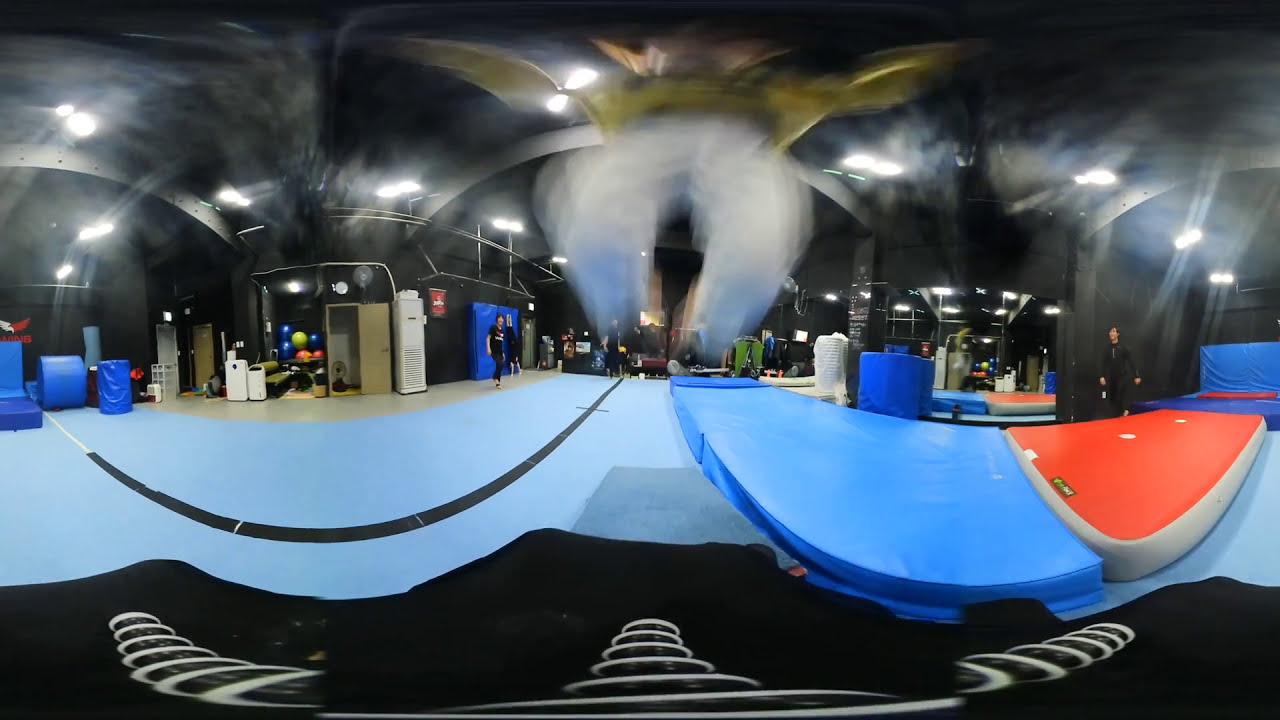The image captures an indoor gymnasium or play course, characterized by an array of blue and red mats organized in a straight line, likely for jumping or playing activities. The walls and ceiling are black, adding to the vivid contrast of the colorful mats. In front of the camera, there's a peculiar overlay effect, possibly resembling the view through a pair of glasses with a gold top and mismatched blue and black frames. This overlay affects the clarity, giving a somewhat blurred, black-and-white impression on parts of the image. To the right, an orange mat with a tan side and adjoining light-blue and dark-blue mats are visible, further adding to the vibrant mix.

In the center of the composition, a man in white pants and a yellow shirt is captured mid-air with his arms outstretched, suggesting he might have just bounced off a trampoline, though it's unclear precisely what he is jumping on. Surrounding him, other people can be seen walking in areas adjacent to the mats, presumably watching his activity. The background reveals a wall lined with additional rolled-up mats, opened lockers, and shelves holding colorful items like blue, green, and red balls. Among the array of soft landing areas, a red board and a black board are also notable, contributing to the dynamic environment of the gymnasium.